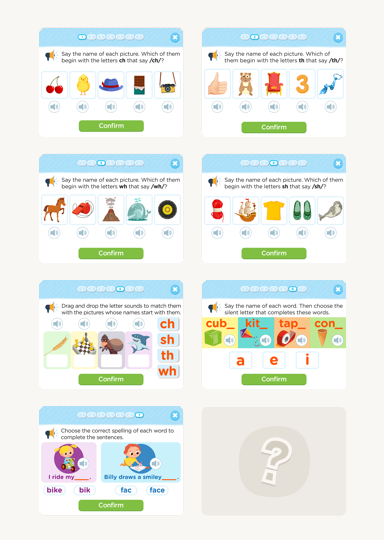This screenshot showcases an English phonetics app designed to help users enhance their pronunciation and understanding of phonetic symbols. The interface displays eight activities or questions, labeled numerically from 1 to 7, with an eighth activity marked by a question mark. Each activity is represented in a compact form, presumably selectable by the user.

One specific activity asks users to "say the name of each picture" and identify which one starts with the phonetic sound represented by the symbol "CH." The question is visually supported by images of a cherry, a chick, a hat, a bar of chocolate, and a camera. Next to each image, there are small audio buttons that, when pressed, play the pronunciation of the depicted item. This auditory feature reinforces phonetic learning by allowing users to hear and practice the correct sounds.

Additionally, a green "Confirm" button is present to submit answers or validate the user’s selections. This module, like others in the app, emphasizes correct spelling and accurate pronunciation of English phonetic sounds, making it a valuable tool for language learning and improvement.